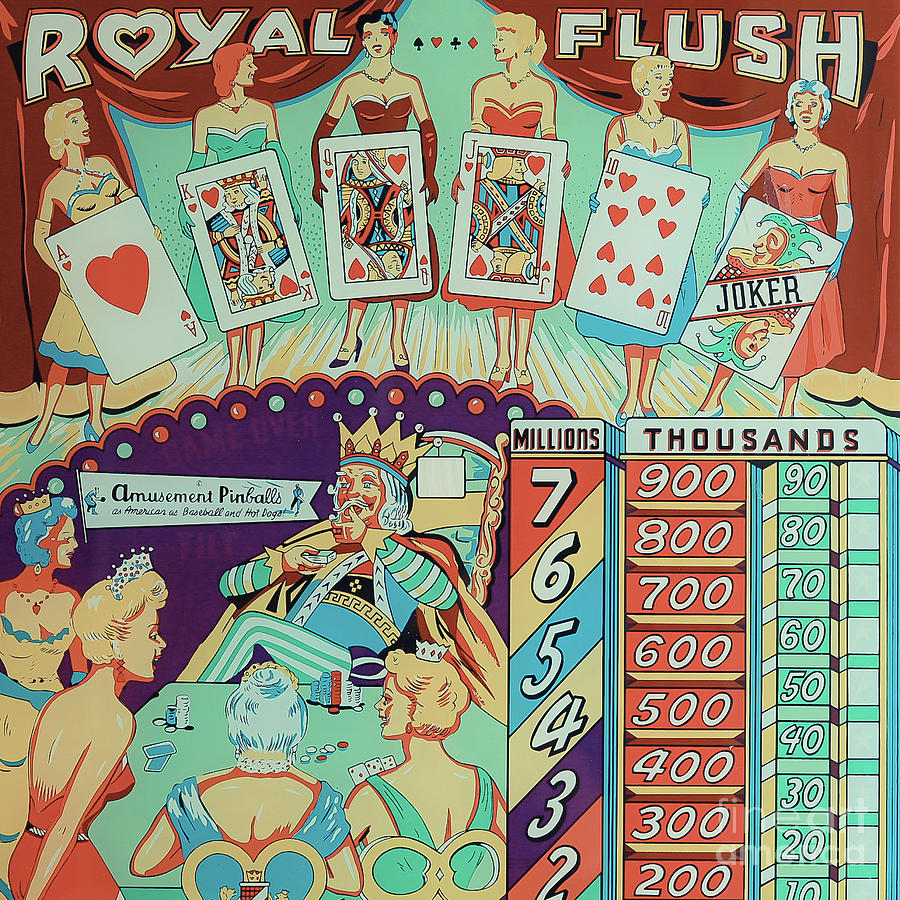This vintage-style pinball machine poster is for the Royal Flush machine and features a vibrant, old-fashioned cartoon design. At the top, the title "Royal Flush" is prominently displayed, with the 'O' cleverly shaped like a heart. The central illustration shows six women, each elegantly dressed in short, strapless dresses and holding playing cards that together comprise a Royal Flush: Ace, King, Queen, Jack, Ten of Hearts, along with a Joker. Below them, a scene depicts a regal king leaning back in a chair at a poker table, surrounded by four women engaged in a game of poker. The king is notably depicted with a towering stack of poker chips. Adjacent to this poker table scene is a detailed scoreboard, segmented into columns labeled "millions" and "thousands," displaying numbers from seven million to two million, and from nine hundred thousand down to two hundred, respectively. A small pennant flag beneath the table reads "amusement pinballs," adding a touch of nostalgic charm to the poster.